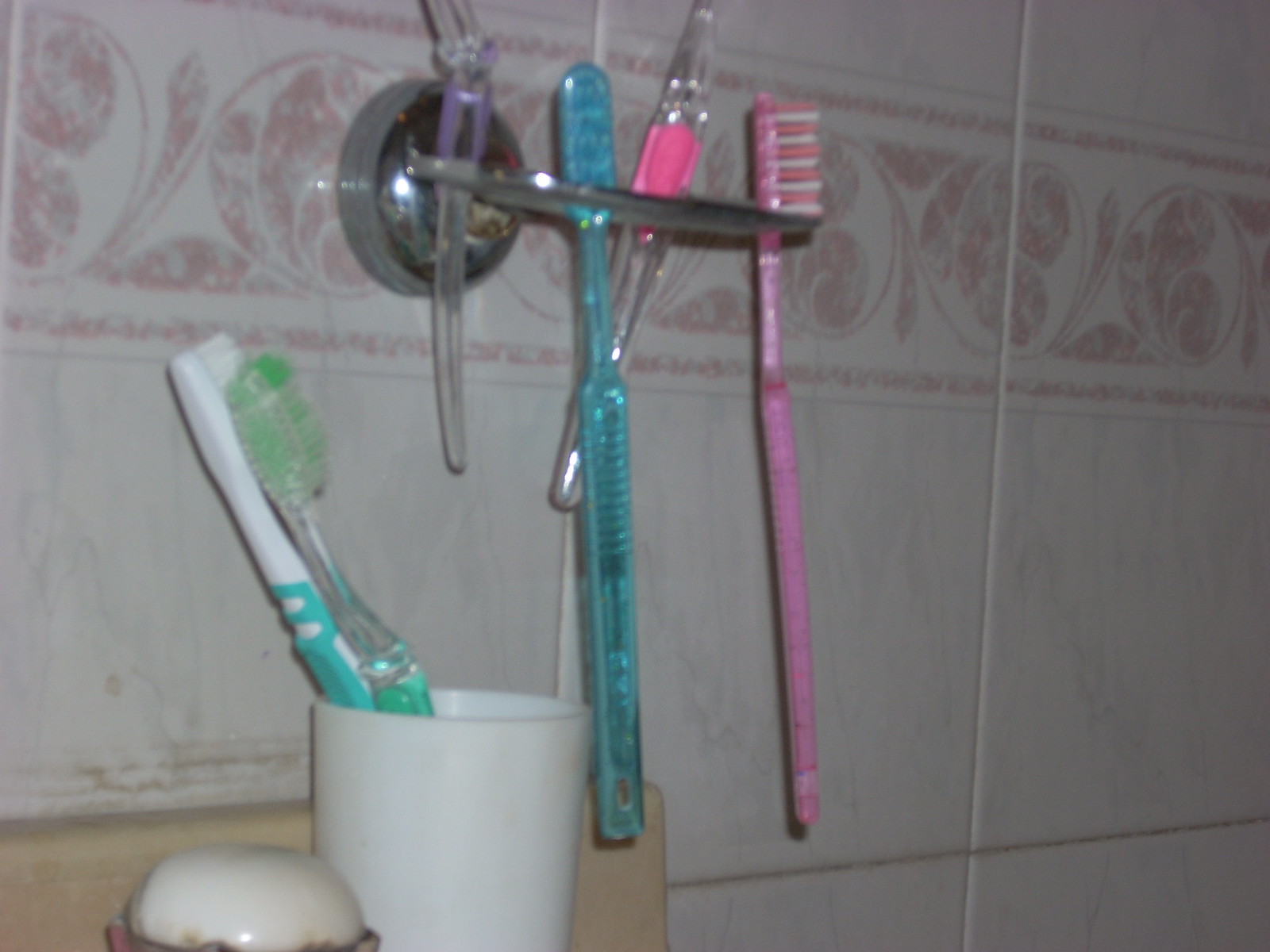In the image, we see a detailed close-up of a bathroom wall adorned with off-white and gray tiles, accented by a decorative strip featuring peach and white patterns. Affixed to the tile wall is a silver metal toothbrush holder, holding four toothbrushes: a clear one with a pink marking, a clear one with a purple marking, a blue one, and a predominantly pink one. To the left on the beige bathroom vanity and backsplash, there is a white ceramic cup containing two more toothbrushes—one clear with a green marking and the other white and turquoise with strikingly white bristles. A bar of soap rests in a soap dish on the sink. The image composition suggests this scene is likely above a bathroom sink in a home, providing an organized and tidy display of variously colored toothbrushes.